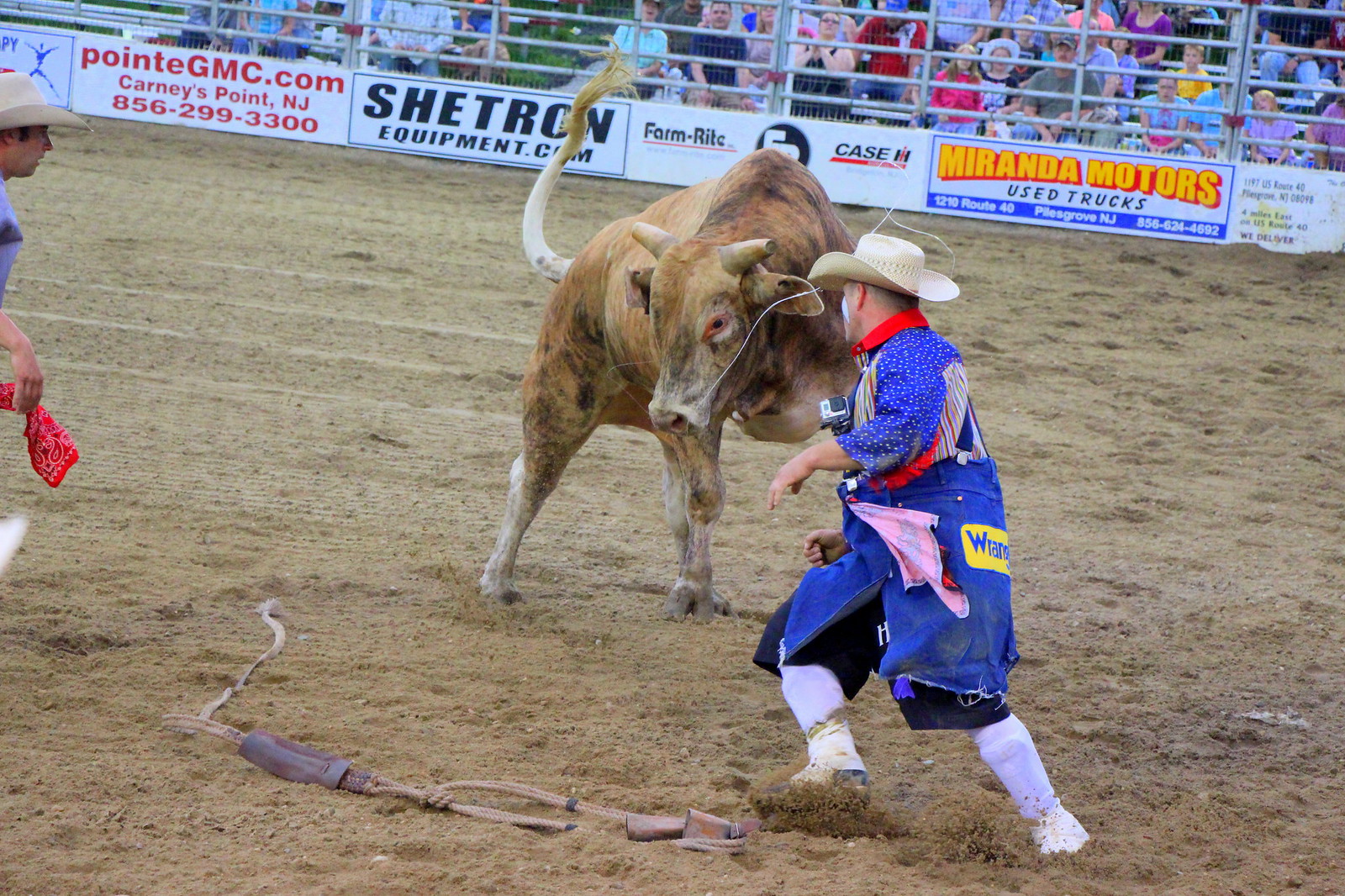In this detailed image of an outdoor rodeo event, there is a brown bull with black spots and shaved horns, standing aggressively in the center of a dirt arena, about to charge at a rodeo clown right in front of him. The clown, dressed in a blue shirt with a red collar, denim overalls, white boots, and a cream-colored cowboy hat, has "Wrangler" emblazoned on the back of his outfit. His face is painted with clown makeup, typical for distracting the bull. 

To the bull's left, approximately eight feet away, another man with a cream-colored cowboy hat and a red bandana is holding a red kerchief, likely to attract the bull's attention. The scene is bathed in diffused daylight, indicating an overcast sky. 

In the background, behind a tall fence designed to contain the bull, an audience can be seen seated in the stands. This fence is adorned with various advertisements, including pointgmc.com, Carny Point NJ, Seatron Equipment, Miranda Motors, and more, which not only add to the lively atmosphere but also indicate the location of the event as New Jersey. The overall setting is a vivid depiction of a tense moment in a rodeo, capturing both the excitement and danger of the sport.